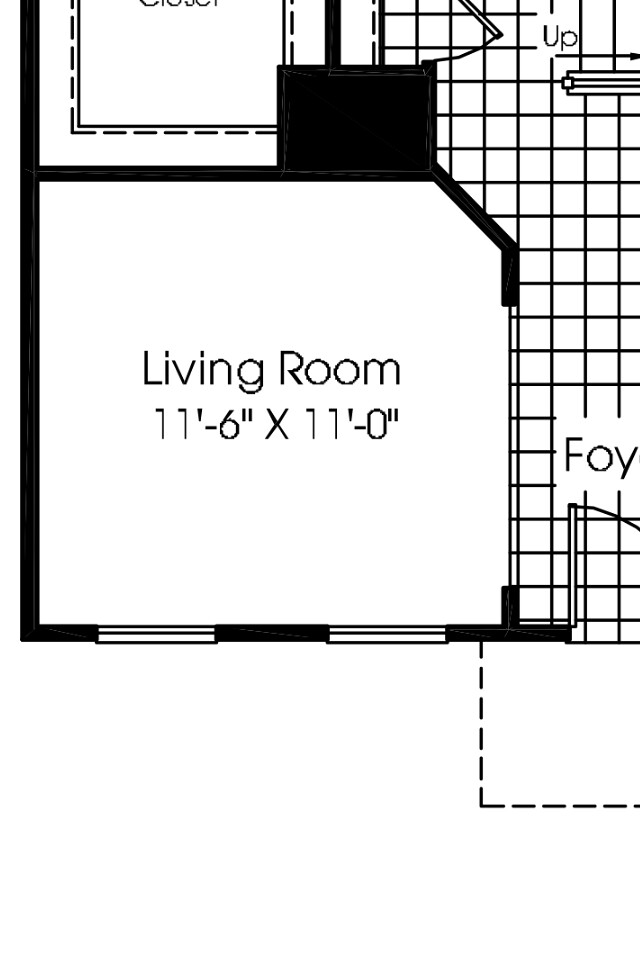A partial scan or screenshot of an apartment blueprint from an internet listing displayed against a white background. The visible section is in black line drawings on white canvas, depicting the lower left corner of the blueprint. The detailed area reveals a square living room labeled 'Living Room' with dimensions of '11'-6" x 11'-0"'. Two dashed lines on the lower left wall signify the presence of windows. A door provides access from the living room to a small space labeled 'FOY', presumably short for foyer, although the term is partially cut off. The foyer features a crisscross black and white pattern and extends to the upper right corner of the visible section. Another room is partially visible in the upper left but its label is cut off, making its identification uncertain.